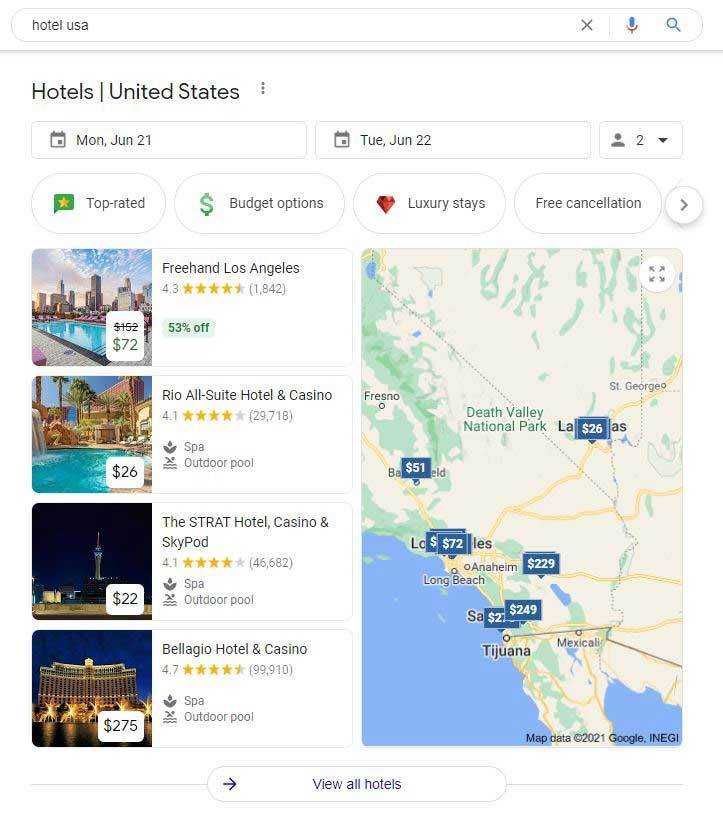This is a detailed screenshot capturing a webpage dedicated to hotel listings in the United States. The background is predominantly white, contributing to a clean and organized layout. At the very top of the page, there is a prominently displayed search bar where the text "Hotel USA" is typed, indicating the search query. To the right of the search bar, there are three buttons: an 'X' button for clearing the search, a microphone icon for voice search, and a magnifying glass icon for initiating the search.

Directly beneath the search bar, a horizontal line divides it from the next section, which starts with the heading "Hotels United States" accompanied by a three-dots menu icon, suggesting additional options or settings.

Further down, there are two date fields showing the check-in date as "Monday, June 21" and the check-out date as "Tuesday, June 22." Adjacent to the date fields is a dropdown menu indicating "2 people," likely for specifying the number of guests.

Following this, there is a set of filter buttons that users can select to refine their search: "Top Rated," "Budget Options," "Luxury Stays," and "Free Cancellation." To the far right of these filters, an arrow icon suggests more filter options can be accessed.

The main content area features four hotel results displayed in a vertical list. Each listing includes a thumbnail image on the left, followed by the hotel’s name and star rating. The hotels listed are: "Freehand Hotel Los Angeles," "Rio All Suite Hotel and Casino," "The Strat Hotel Casino and SkyPod," and "Bellagio Hotel and Casino."

On the right-hand side of the page, a map provides a visual representation of the hotel locations, assisting users in choosing based on geographic preference.

This description encapsulates the layout and elements of the hotel listing page in detail, enabling users to understand its functionality and visual structure without seeing the actual screenshot.